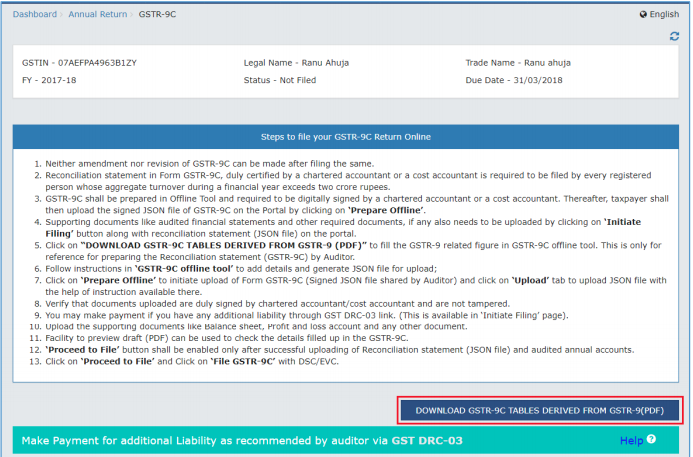The image displays a detailed Dashboard interface for filing the GSTR-9C annual return. At the top, the word "Dashboard" is prominently shown. Below this header, the text "Annual Return" is displayed, followed by "GSTR-9C." On the top right corner, the language preference is set to "English."

In the section below, specific details are listed, including:

- GST Identification Number (GSTIN): 07AEFPA496-3B1ZY
- Financial Year: FY-2017-18
- Legal Name: Rana Auja
- Status: Not filed
- Trade Name: Rana Auja
- Due Date: 31-03-2018

A guide titled "Steps to file your GSTR-9C return online" outlines 13 necessary steps, advising users to:
1. Prepare offline
2. Initiate file
3. Download it
4. Use the offline tool
5. Prepare offline
6. Proceed to file

Further instructions detail the filing process, including the need to download GSTR-9C tables derived from GSTR PDF and make payments for additional liability as recommended by the auditor via GST-DRC-03. A "Help" button is provided for additional assistance.

The interface also features a button labeled "File GSTR-9C" for users to submit their return.